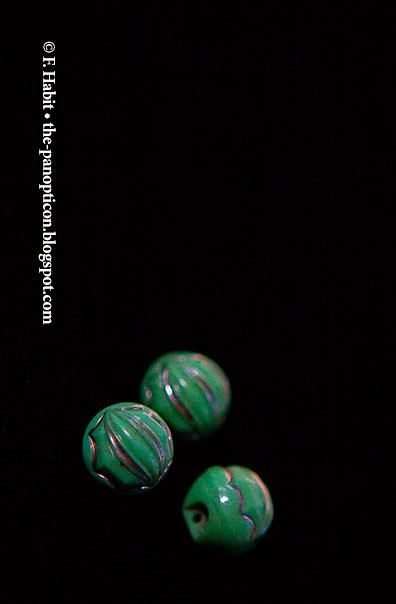The image features a tall vertical black rectangle, rotated counter-clockwise, with the caption "© F. Abbott, thepanopticon.blogspot.com" written vertically along the left side. At the bottom of the rectangle, there are three decorative beads positioned diagonally, extending from the bottom center towards the middle of the image. These beads are green with purple creases and indentations, giving them a striped appearance. The beads are designed for use as jewelry components, like necklace or bracelet beads, with visible holes for stringing. The bead farthest in the background is slightly out of focus. The image appears to be an advertisement for jewelry or accessories.